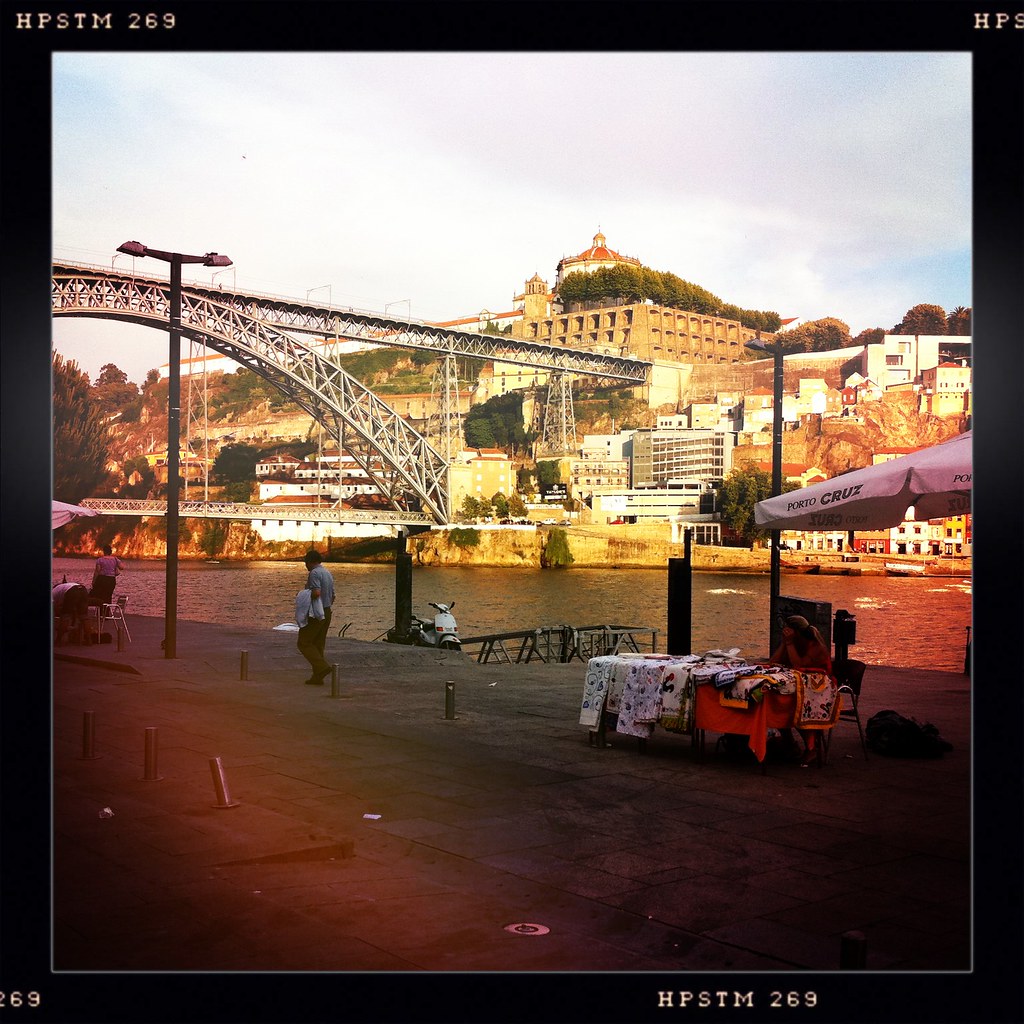The photograph, encased within a black border inscribed with the codes "H P S T M 2 6 9" in the top left and bottom right corners, "H P S" in the top right corner, and "6 9" in the bottom left corner, presents a vibrant cityscape. Central to the image is a grand, metal-framed bridge spanning a wide river, anchored by sturdy towers and girders. On the far side of the river, a hillside rises, adorned with stone buildings, some featuring domed roofs and turrets that evoke an architectural blend of churches and historical monuments.

In the foreground, alongside the river, lies a bustling boardwalk. This area, appearing like a concrete dock, is animated with various activities. Tables laden with products for sale, possibly including blankets, shawls, or shirts, are spread out, one of which is shielded by an umbrella bearing the inscription "Porto Cruz." Nearby, a small motor scooter is parked, and two men can be seen walking. These elements come together to create a scene rich in detail and movement, capturing both the monumental bridge in the background and the lively marketplace in the foreground.